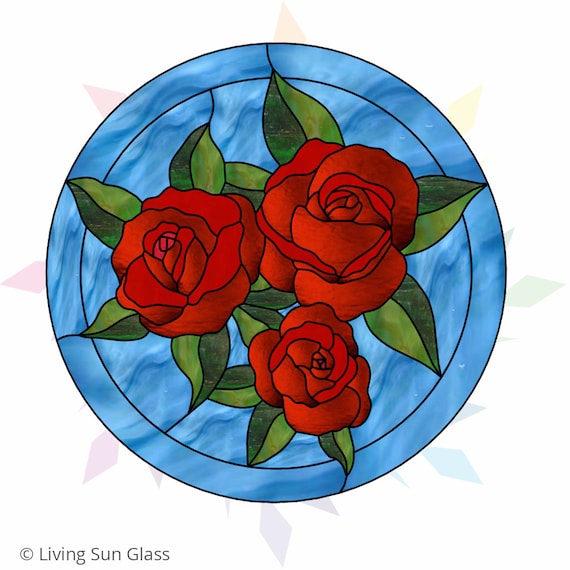This intricate glass art piece, capturing detailed craftsmanship, features a circular design with a striking blue background, enhanced digitally. Dominating the center is a vivid representation of three open red roses, their delicate petals in various shades of red, framed by a series of intricate black outlines. These roses are surrounded by an arrangement of dark and light green glass leaves, each detailed with black borders. The composition further includes a slimmer black circle within the blue round frame, adding depth and structure. The background of the image is off-white, seamlessly blending into a spectrum of faintly colored digital arrows and triangular shapes in purples and orange-reds, projecting outwards. In the bottom left corner, a discreet but clear label reads, "© Living Sun Glass," ensuring recognition of the artwork’s origin.